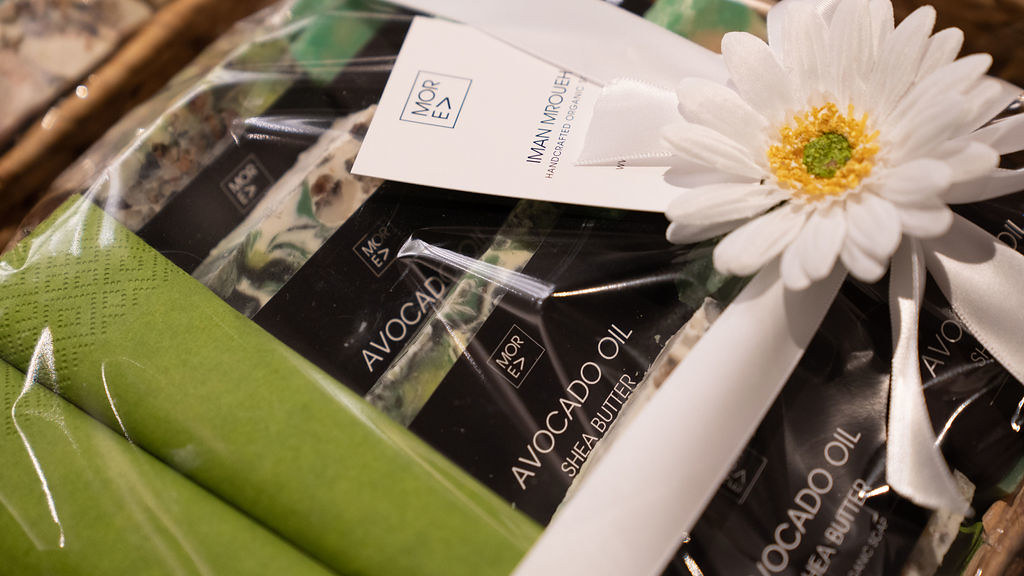This image is a detailed close-up of a gift bag containing an assortment of products. The gift bag features a prominent white banner adorned with a white daisy at the top, which serves as a bow. The daisy's center is highlighted with yellow pollen and green accents, making it a focal point of the presentation. Nestled just behind the banner is a card that reads "More Iman Handcrafted Organic" (with some text obscured), indicating a touch of personalized craftsmanship.

The interior of the bag reveals several goodies, including packets of avocado oil with shea butter. These packets are sheathed in a sleek black packaging topped with white text, and they are neatly arranged and stacked. The entire ensemble is wrapped in plastic, secured with a white ribbon tied in a bow, which features the aforementioned daisy at its center.

To the right of these products, there is a piece of green fabric or paper towel with a decorative border, adding an additional layer of elegance to the presentation. All of this is seated inside a brown basket, making it a well-organized and visually appealing gift.